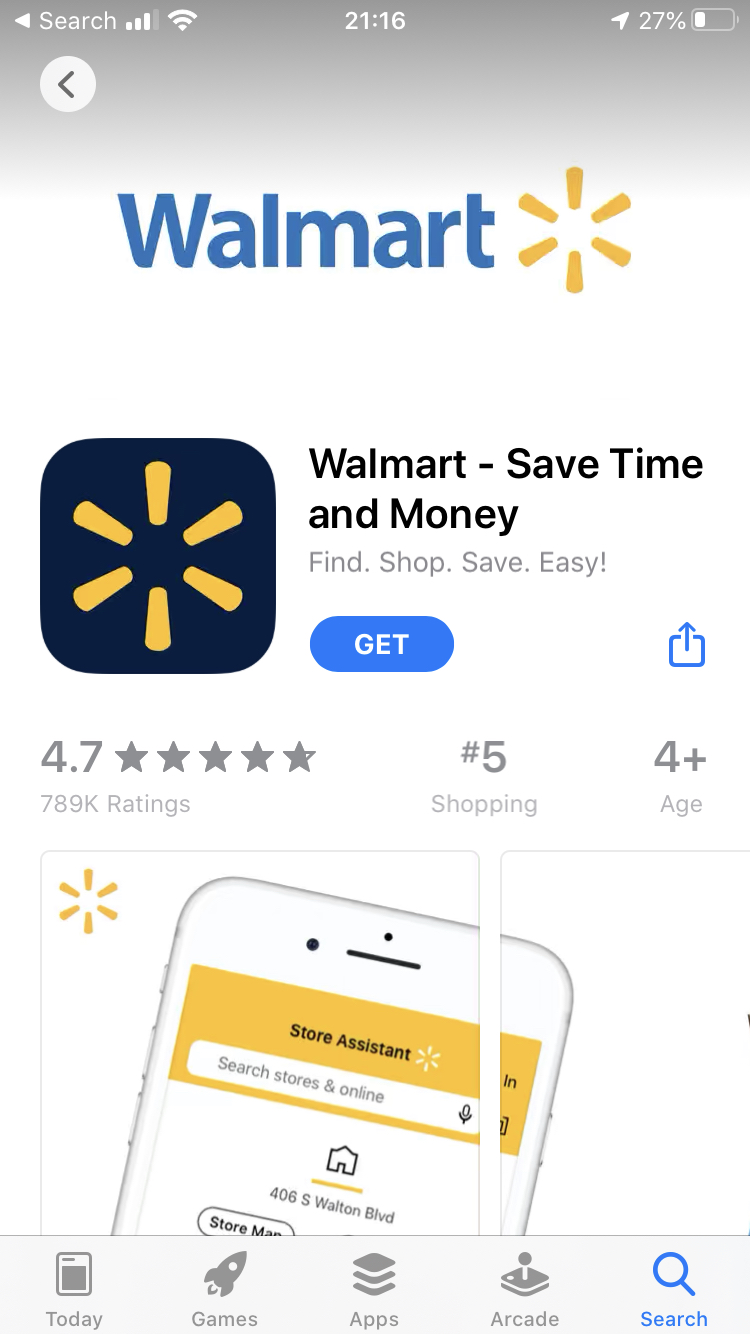Screenshot showing the Walmart App Download Page

In this screenshot taken from a cell phone, the user interface displays the Walmart app download page. At the very top, there is a status bar with the following: a 'search' label on the upper left, a Wi-Fi symbol, the time displaying "21:16" in the center, and a battery indicator showing 27% on the upper right.

Just below the status bar, the page primarily features a predominantly gray-to-white gradient background. In the upper center, the word “Walmart” appears in blue typography accompanied by a yellow sunburst-like logo next to it. Further down, there is a small black, rounded square icon showcasing the Walmart logo in its center.

The main body contains descriptive text stating “Walmart – Save time and money. Find, shop, save easy.” Below this, a prominent blue oval button labeled “GET” indicates how to download the app. Accompanying this information, it rates the app 4.7 out of 5 stars and specifies that it is the #5 shopping app suited for ages four and up.

The lower section of the screen displays an illustration of a smartphone with features like “store assistant” and “search stores.” Finally, a navigation bar at the very bottom lists different sections such as “Today,” “Games,” “Apps,” “Arcade,” and “Search.” The "Search" icon is highlighted in blue, while the other options are gray.